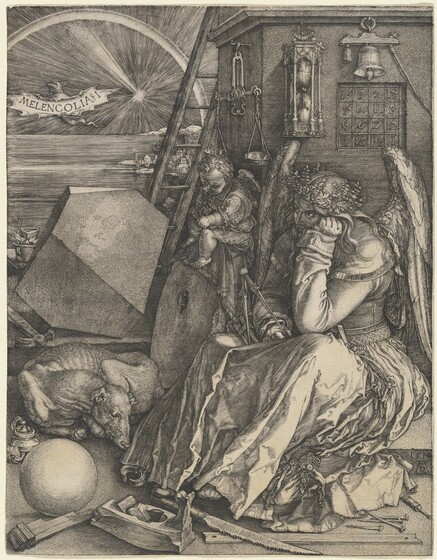In this intricate and melancholic medieval black and white drawing, a pensive angel sits on the floor of a cluttered room adorned in a long flowing robe. The angel's long hair cascades down their back, partially obscuring large wings that poke up prominently. One hand rests thoughtfully on the angel's cheek while the other lightly holds a pen or scepter. At the angel's feet lie a sword and a sphere, with a pig curled up to the left. 

A cherubic figure with delicate wings hovers near the angel’s right shoulder, adding to the scene's somber atmosphere. Background details reveal a richly detailed interior space scattered with what seems like a sprawling collection of objects, including pillows, cloth, and a weighing scale. 

A building with a bell, window, and ladder dominates the back, suggesting a deeper symbolic meaning. Sun rays pierce through the background, casting light on the wall where letters spell out "Melancholia." This word, along with the desolate expressions of the angel and cherub, heightens the overall mood of deep introspection and sorrow.